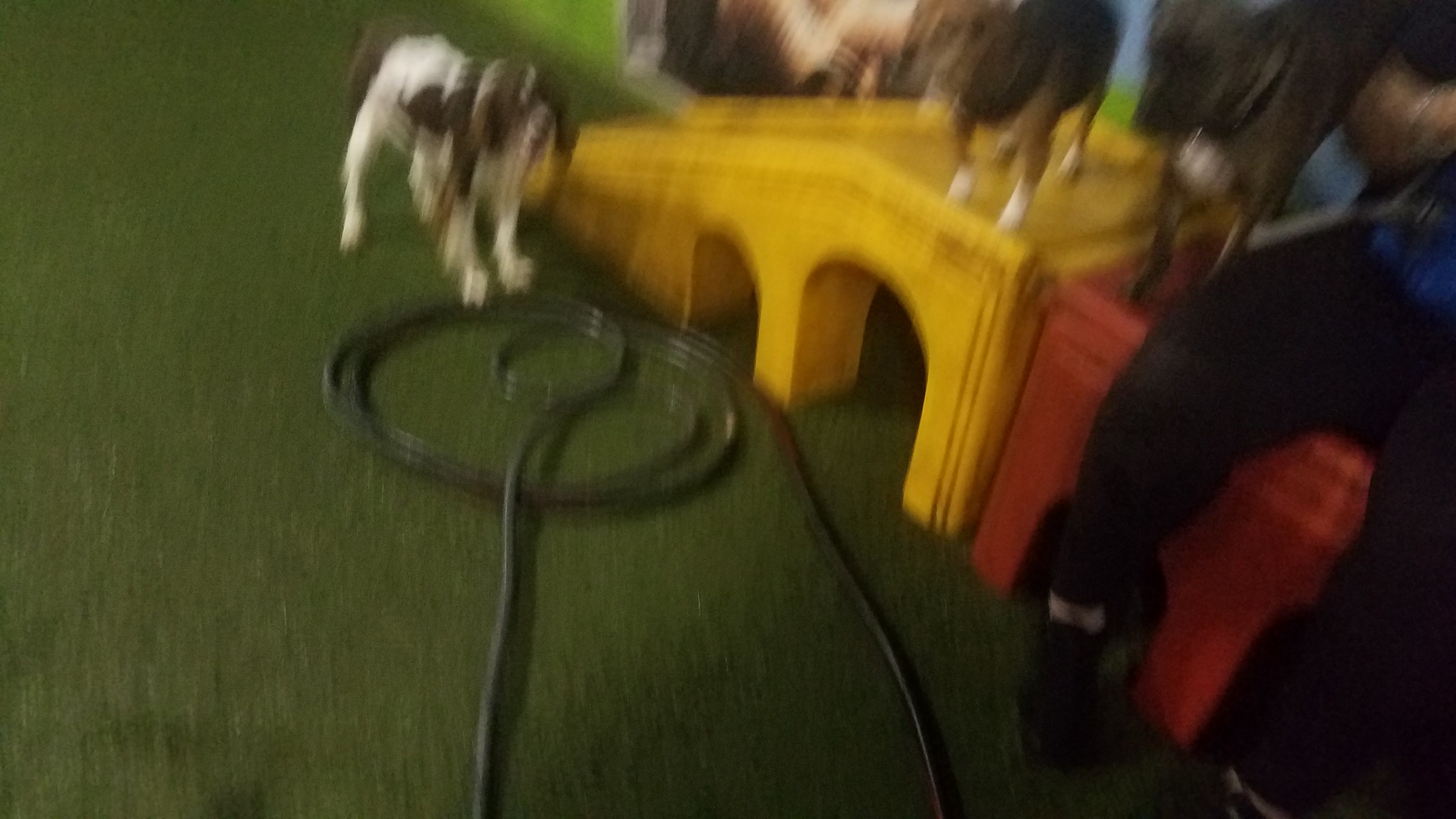This photograph captures a vibrant scene from a dog park event, set on a meticulously manicured green turf. A green hose winds across the scene, creating loops in its path. In the center, a person dressed in black pants sits on a red plastic box. Adjacent to the box is a bright yellow slide with arch-shaped cutouts on the sides, leading down to the ground. Two brown dogs are standing on the yellow and red platforms, exploring their elevated positions. To the left, a white and brown dog, with its legs predominantly white and its body and face primarily brown, observes the scene attentively.